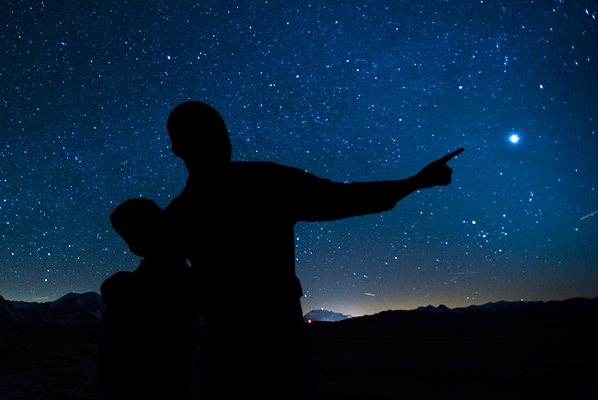The photograph captures a stunning night sky with a myriad of stars and possibly planets, set against a vibrant dark blue and crisp black backdrop. Towards the bottom of the image, the horizon subtly transitions into a silhouette, tinged with faint hues of orange and yellow, suggesting distant city lights or a setting sun. Prominently featured are the shadowy outlines of an adult, possibly a bald man, holding a child, who might have short hair. The adult is pointing with his right index finger toward a particularly bright celestial object, which could be a planet or a large star, in the middle right of the image. The scene conveys a sense of awe and wonder, with the vastness of the universe contrasted against the intimate moment of stargazing.